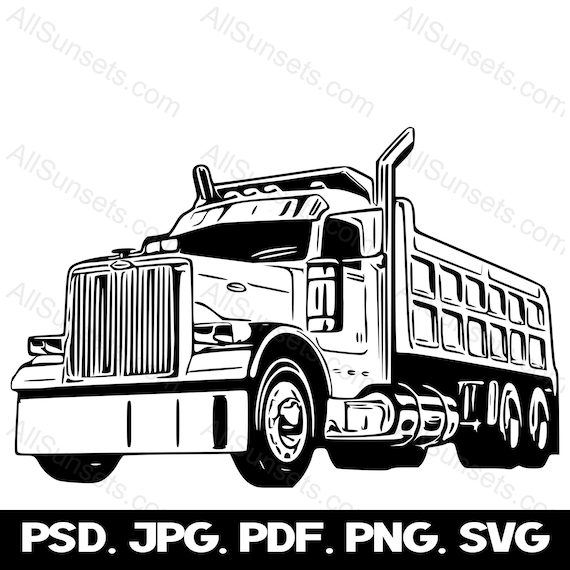This detailed illustration, in black and white, depicts a dump truck rendered in a mix of comic and realistic styles. The truck is shown from a side-angled perspective and features six wheels, including double wheels at the rear, and a prominent front grill. It is equipped with two large smokestacks at the front. Notably, the dump truck's cargo area is designed with six panels on both the top and bottom. The windows of the truck are blacked out, and there is deep shading underscoring the truck and its wheels, emphasizing the illustration's depth. The image is overlain with a watermark that reads "allsunsets.com" in a diagonal pattern across the truck. At the bottom of the image, a black banner with white, capitalized text displays the file formats "psd.jpg.pdf.png.svg."